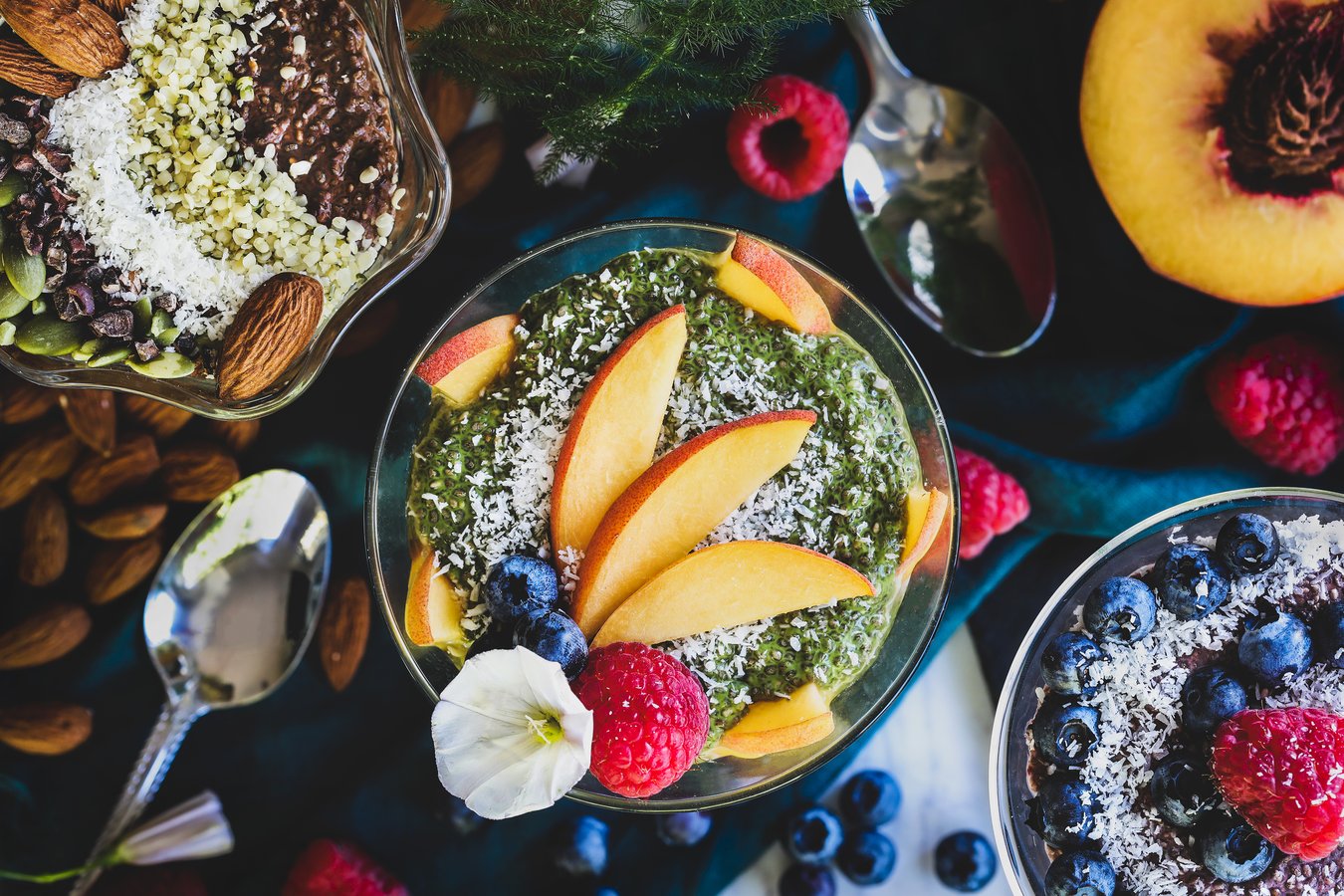The photograph captures a vibrant, festive meal set on a table laid with a blue tablecloth. Dominating the scene are three distinct glass bowls, each artfully curated with an assortment of toppings and garnishes. The bowl on the left, a wavy star-shaped design, features a mix of what appears to be oatmeal adorned with pumpkin seeds, chocolate shavings, grains, shredded coconut, and scattered almonds. 

In the center, the primary focus is a circular bowl filled with creamy yogurt or tapioca, lavishly topped with fresh peach slices, a raspberry, two blueberries, and a vibrant green pesto-like substance. This bowl is further garnished with a sprinkling of shredded coconut and delicate white flowers, enhancing its visual appeal.

To the right, another circular glass bowl showcases layers of blueberries, shredded coconut, and a central raspberry, meticulously arranged. Scattered almonds and blueberries embellish the table, adding to the rustic charm. Silver spoons are strategically placed, with one reflecting the photographer, subtly hinting at their presence. The overall setting, complete with a mix of fresh fruits like raspberries, half a peach, and accents of potpourris, creates an inviting and picturesque dining experience.